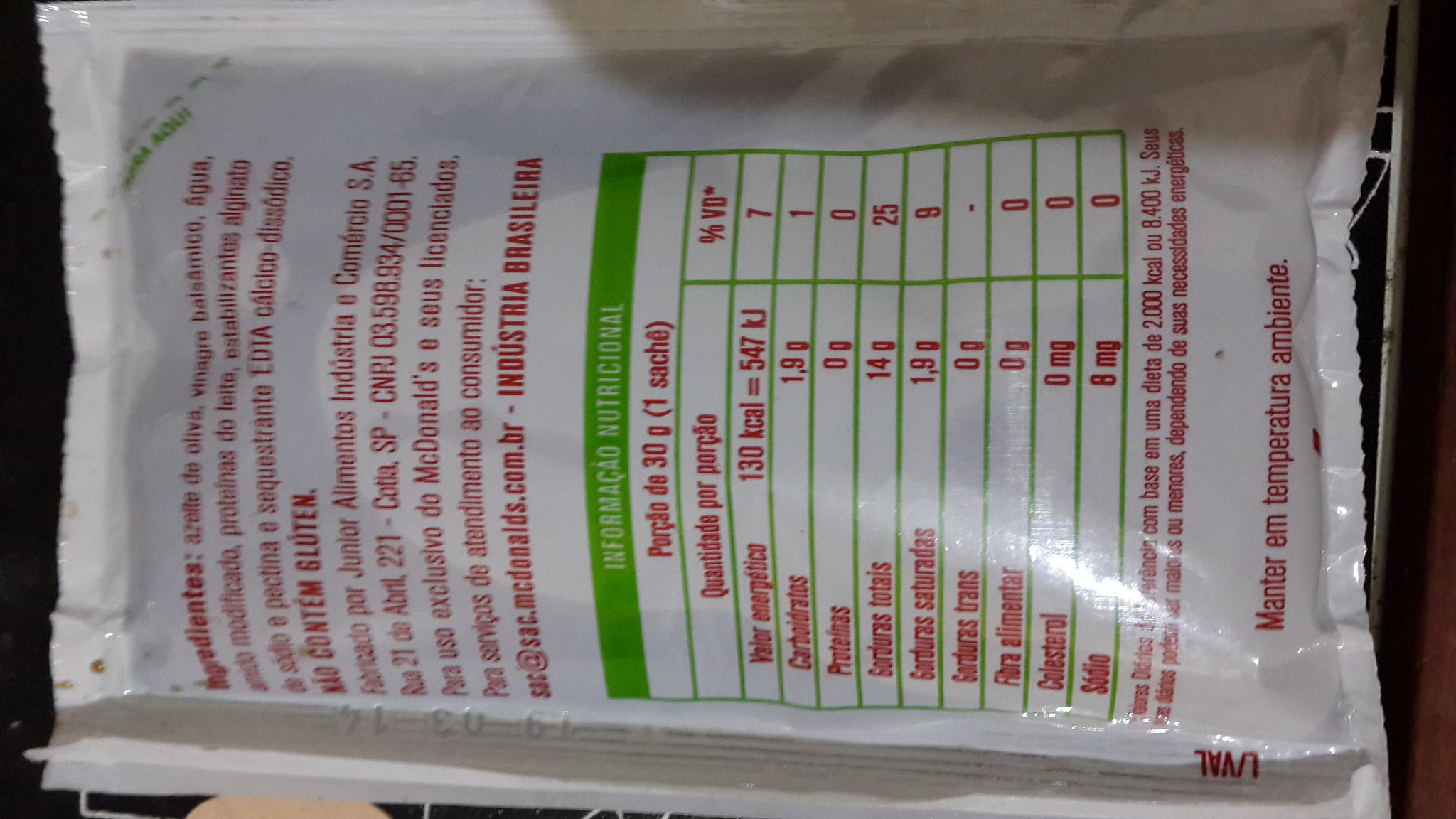The image features a zoomed-in view of a white packet, showcasing its nutrition label, which is oriented sideways and possibly written in Spanish. At the top of the label, on the left-hand side, there is a paragraph of red text. Directly below this paragraph starts the nutrition information, marked by a green bar, with the details presented in a green, chart-like format, also in red text. Below this nutritional information is additional red text. The entire image is framed by a narrow black background on the left side and a slightly wider dark brown area on the right.